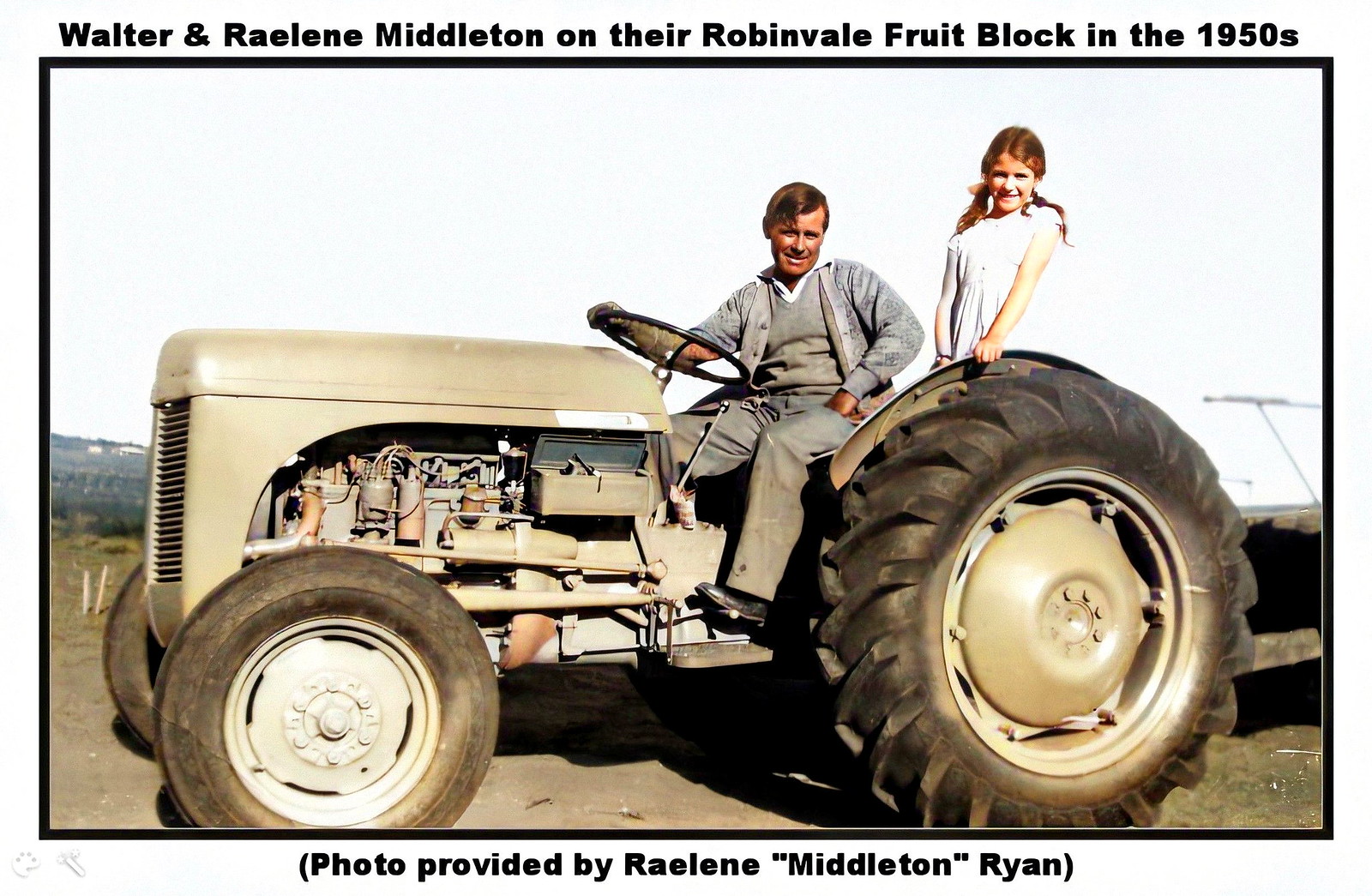In this aged color photograph from the 1950s, we see a man named Walter Middleton and a young girl named Raylene Middleton on their Robinvale fruit block. The composition captures a side profile of a large, green tractor with a small front wheel and a large rear wheel, surrounded by a dusty field. Walter, appearing somewhat sunburned, is dressed in dusty slacks, a gray suit coat over a sweater vest, and a white shirt. He is seated at the tractor's steering wheel, his gloved right hand gripping it. Beside him, towards the rear of the tractor, stands Raylene, who looks about 11 years old. She is wearing a white dress and has red hair styled in pigtails, holding onto the tractor with one hand. The scene is framed by text at the top that reads, "Walter and Raylene Middleton on their Robinvale fruit block in the 1950s." At the bottom, it is noted, "Photo provided by Raylene Middleton Ryan." In the background, mountains loom behind sparse trees, completing the nostalgic and detailed rural scene.